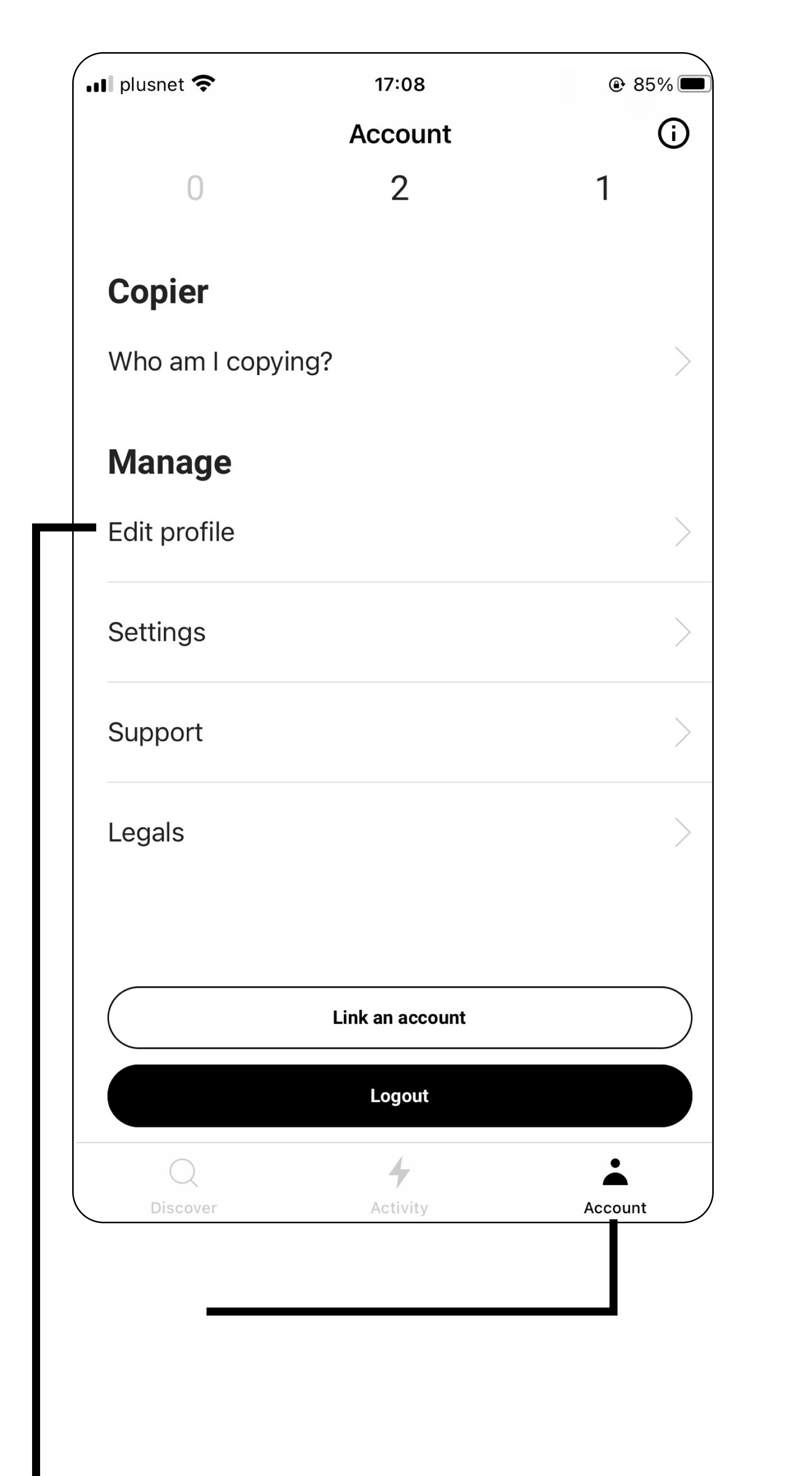The screenshot shows a mobile interface displaying the PLUSNET network at the top with a 17:08 timestamp and an 85% battery level. Below the header, the interface features a status count reading "0, 2, and 1" next to an "i" icon inside a circle. The screen lists options such as "Manage," "Edit Profile," "Settings," "Support," "Legals," followed by a white rectangular button labeled "Link an Account" with the text in black. At the bottom, there's a black rectangular button labeled "Logout" with white text. Navigation icons are positioned at the footer displaying "Discover" with a magnifying glass icon, "Activity" with a thunderbolt symbol, and "Account" with a profile icon. The "Account" section is highlighted in black, while the "Discover" and "Activity" sections are greyed out.